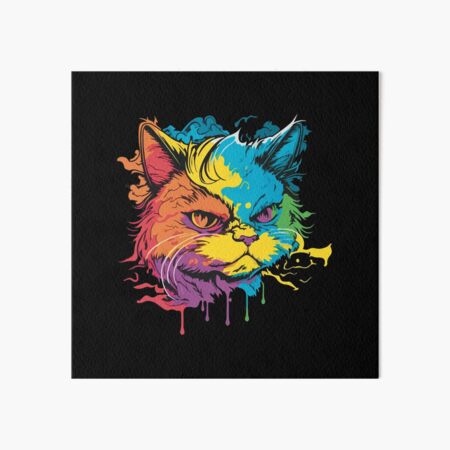This image features a stylized rendering of a cat’s head, centered within a black background. The artistic style merges graphic design elements with urban graffiti aesthetics, resulting in an avant-garde and psychedelic appearance. The cat has a general look of anger or annoyance, its expression accentuated by its perky ears. Multi-colored drips and splashes create a vibrant and dynamic effect. The color palette includes purple, orange, yellow, brown, green, white, and blue. Specific color details include: one eye in orange with the other in purple, yellow around the nose, purple along the mouth, and a mixture of red, blue, and yellow on the ears. The top right of the cat’s head features bright blue, while the left ear is layered in red. Purple covers the bottom right of the face while the bottom left drips with yellow and green. This dripping effect enhances the overall uniqueness and creates a sense of movement within the piece.